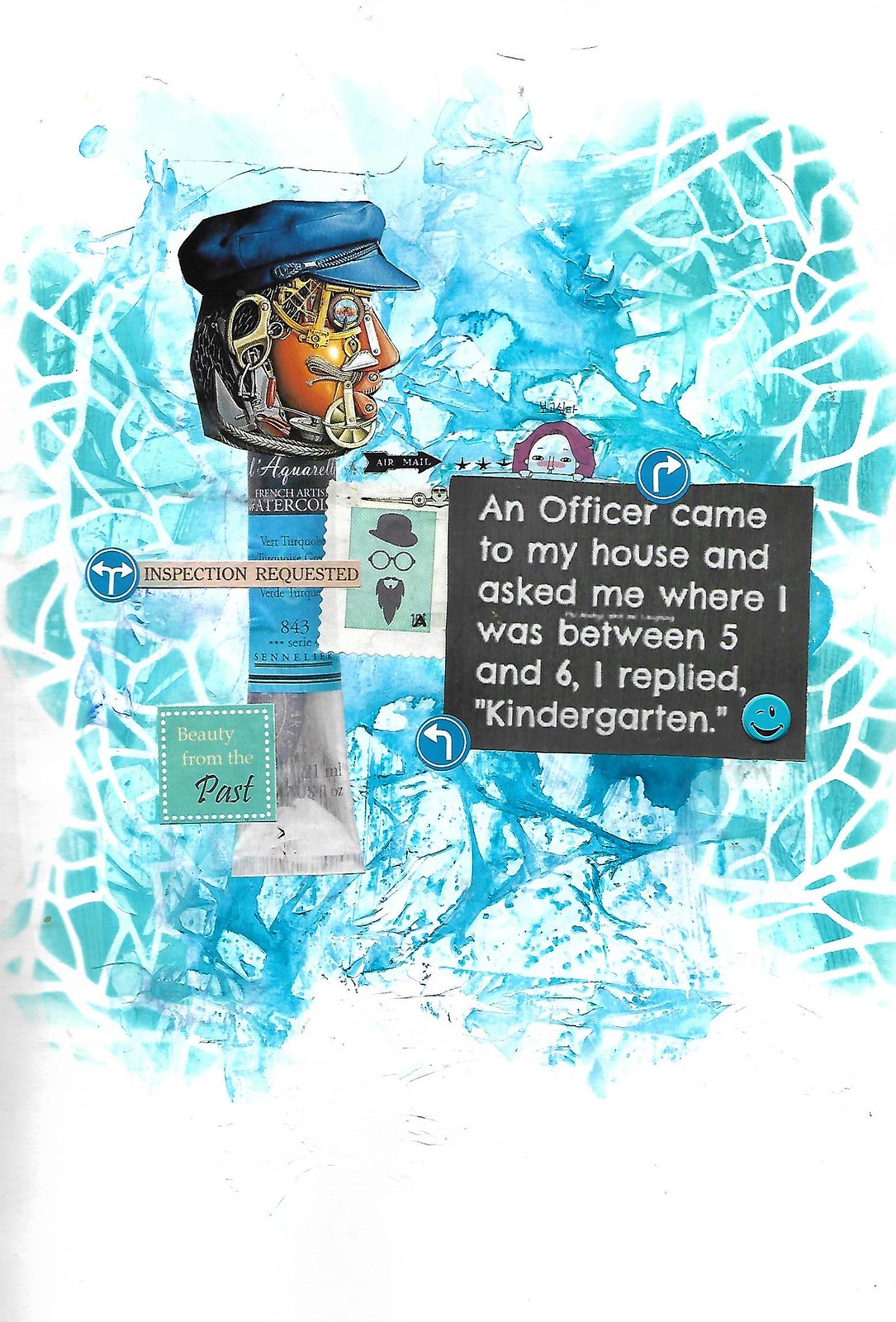The image is a complex artistic collage featuring a blue, icy blue, and turquoise background, reminiscent of a cracked watercolor effect. Dominating the composition is a side profile of a drawn figure wearing what appears to be a blue hat, similar to a captain's or policeman's hat, positioned on the left side. The figure's head is filled with a variety of objects, including a fishing net, a wheel, and a knife, creating an intricate and thought-provoking visual. To the right of the figure, there is a gray box with white text that reads, "An officer came to my house and asked me where I was between 5 and 6. I replied, kindergarten." This humorous text is accompanied by a blue, winking smiley face. Additionally, there is a stamp-like image with white borders and an aquamarine square inside, featuring illustrations of glasses, a beard, and a hat, disconnected from any discernible profile. Another turquoise square contains the phrase "Beauty from the past," adding to the collage's enigmatic and somewhat random feel.